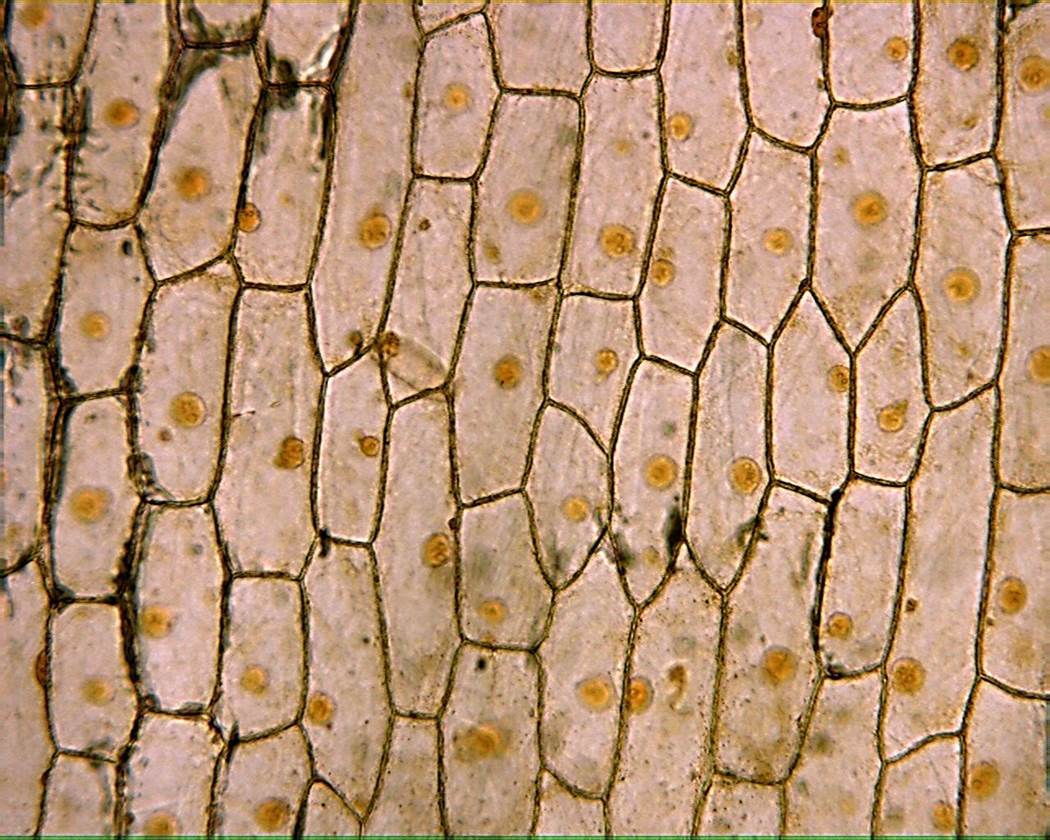This detailed microscopic image reveals an intricate honeycomb-like pattern, with each hexagonal cell housing a vibrant orange circle filled with bubble-like structures or possibly smaller cells. The cell walls are defined by dark brown lines, creating a stark contrast against the lighter, tan-colored elements within each section. Notably, in the upper left corner, the dark brown lines appear slightly smudged, extending down the left side of the image. Additionally, similar smudging is observed towards the middle right section. Black specks are scattered around the lines on the middle bottom right side, adding another layer of complexity to the visual landscape.